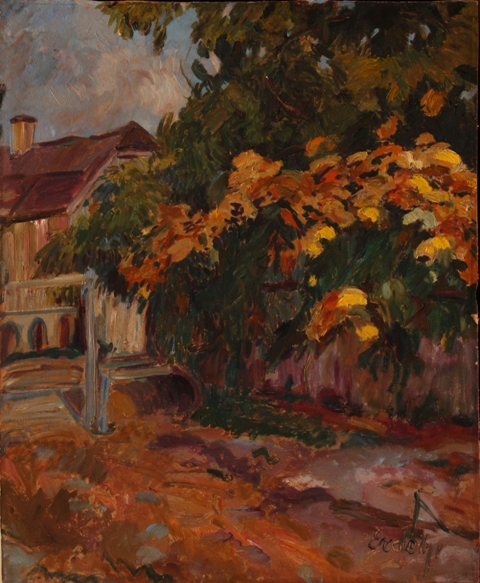This colorful impressionist artwork, possibly created in the late 19th to early 20th century, is most likely done in watercolor or oil paint. It vividly captures a serene countryside scene. Central to the composition is a charming country house on the left side of the painting, identifiable by its brown color and dark brown roof, along with a chimney. The house is accompanied by what seems to be an elevated walkway with arches for passage underneath. 

In front of the house, there is a vibrant meadow, rich with diverse hues of orange, green, and patches of purple flowers. A dirt path winding through this meadow leads up to a gate, suggesting an entrance to the property. To the right of the house stands a prominent large tree with leaves that range in color from green to yellow and brown, adding texture and depth to the scene. 

In the background, a magnificent blue sky with white clouds stretches above, while the upper right corner of the painting is adorned with detailed tree foliage. Additionally, there's a light pole with a fixture on the left-hand side towards the mid-range, contributing to the rural charm of the painting. The lower right corner of the painting features an artist's signature, although it is difficult to decipher.

This painting skillfully combines elements of natural beauty and rustic architecture, all rendered in the distinct, loose brushwork characteristic of the impressionist style.